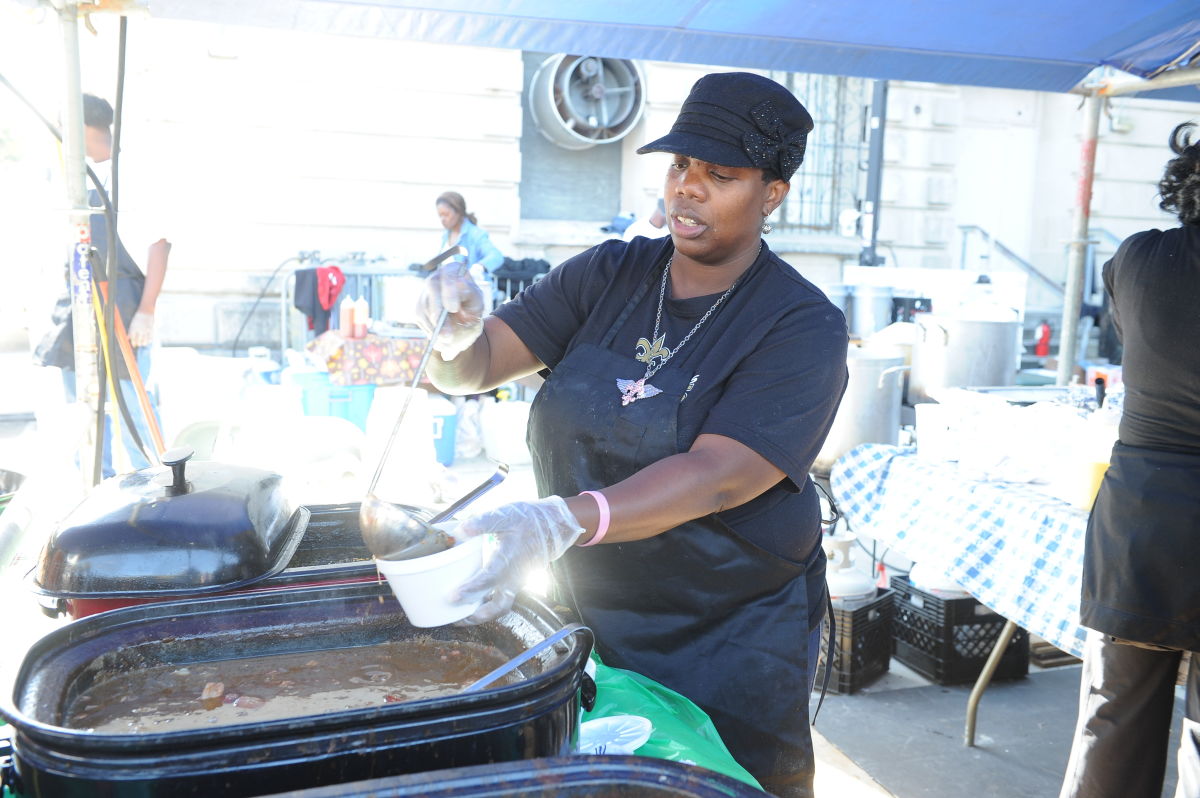The image depicts an outdoor event under a blue tent, with white poles visible in the upper corners. The background features a slightly blurred older building with a protruding window unit fan and indistinct people milling about. In sharp focus at the center is a heavyset woman deeply engrossed in preparing a dish, likely a stew or gumbo. She is dressed in a black baseball cap adorned with a black ribbon, a black t-shirt with a New Orleans Saints logo, and a black apron. Around her neck hangs a distinctive necklace with a wing-shaped pendant in blue and red. She wears plastic gloves for food handling and is seen ladling the stew into a white bowl from a large, black rectangular crock pot. Her right hand holds the ladle while her left hand steadies the bowl. Checkered blue and white tablecloths cover the tables around her, and the partially cropped figure of another worker, dressed similarly in black, is visible in the background, with her back to the camera. The entire scene is well-lit, adding a bright, white hue to the distant background.